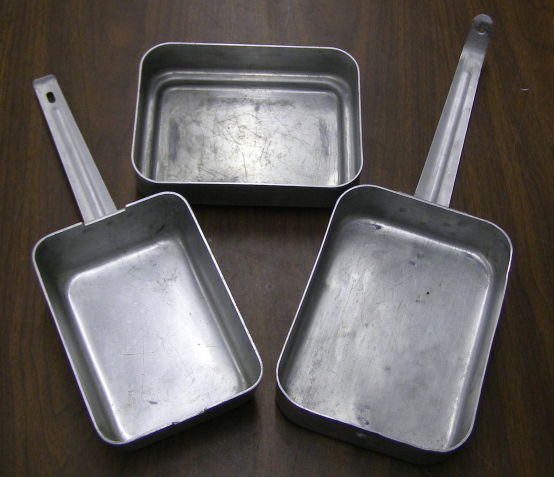The photograph is a top-down, slightly angled view of three metal cookware pans positioned on a dark oak wooden surface. The wood grain, which exhibits a light black pattern running from the back to the front, adds a rustic touch to the scene. 

In the background, there's a deep, rectangular pan with rounded corners that has a double ridged bottom. This back pan is aligned horizontally, with its longer side parallel to the top edge of the image. In the foreground, two smaller, similarly shaped pans—both rounded rectangles—are positioned diagonally. They feature long metal handles that extend backward at 45-degree angles, forming a V-shape. 

All three pans possess a weathered, old-fashioned appearance, which suggests they have been used extensively over time. While the rectangular pan at the back lacks a handle, the two foreground pans are equipped with sturdy, utilitarian handles. The overall composition and aged aesthetic of the pans hint at their potential versatility, possibly in baking, cooking, or other culinary applications.